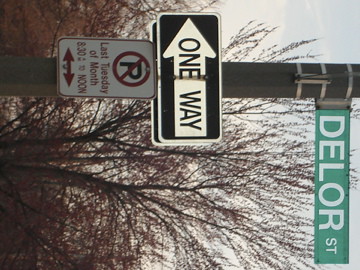The image is a horizontal rectangle that appears to have been rotated 90 degrees clockwise, originally taken in a vertical perspective. It depicts a trio of road signs affixed to a gray pole about 6 inches wide, which extends from the top to the bottom of the image. The primary street sign at the top is green with white text, reading "Delore Street." Beneath it, there is a black One Way sign with a white arrow pointing to the left and white text. Further down the pole, a No Parking sign is visible, displaying "Last Tuesday of the month, 8:30 to noon" in red text on a white background, with arrows pointing both left and right. The background features a light blue sky with some white clouds, indicating a sunny day. Surrounding the signs are trees and bushes, devoid of leaves, suggesting the image was taken during winter.